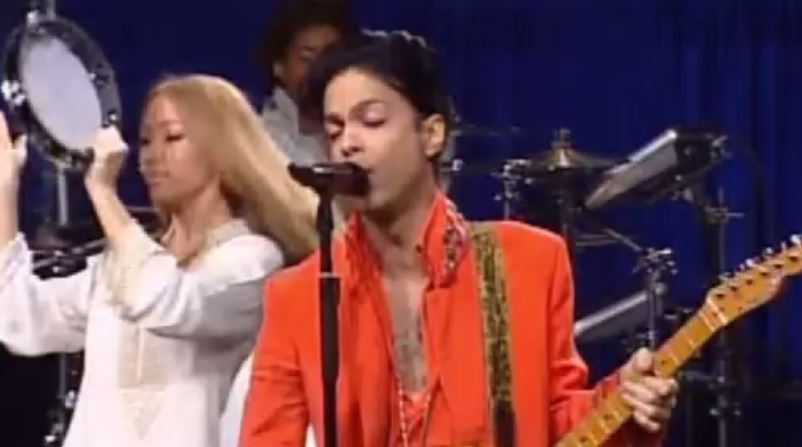The image captures a blurry screenshot of a live performance by the artist Prince, positioned centrally in the photo, which is formatted in a horizontally oriented rectangle. Prince is singing into a black microphone on a stand, his eyes closed, with his mouth slightly open. He wears a coral-colored open jacket, revealing his bare chest adorned with orange or pink beads, and holds the neck of a brown guitar, supported by a light brown guitar strap. His hair is black and free of facial hair. Behind Prince, slightly to his left, stands a woman with long honey-colored hair and very light brown skin, dressed in a long-sleeve white top, playing a white tambourine with black edges. Further in the background, a dark-skinned drummer wearing a white shirt is partially visible behind a drum kit. The backdrop features a deep blue curtain, enhancing the intimate ambiance of the performance.